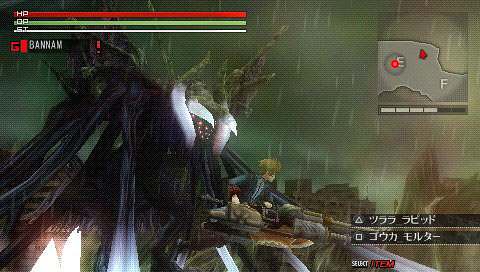**Caption:**

In this vibrant screenshot from a video game, several user interface elements and in-game visuals are present. On the upper left corner, the score information is displayed, showcasing a horizontal bar with segments in red, green, and white extending to the middle of the screen. This bar is labeled "HPOP." Below this, the name "Banham" appears, preceded by a prominent red letter 'G' and a vertical red line.

The central focus of the image features a tree-like creature, adding a fantastical element to the scene. Positioned in the middle bottom, a young boy with blonde hair and striking blue eyes is seen. He wears a blue jacket with a white stripe down the center and is holding a large, futuristic-looking gun in front of him. 

In the upper right corner, a mini-map indicates his location within the game. Towards the lower right corner, Chinese characters provide additional information, contributing to the game's immersive and diverse environment. The intricate detailing and the layering of UI elements convey a rich, interactive gaming experience.